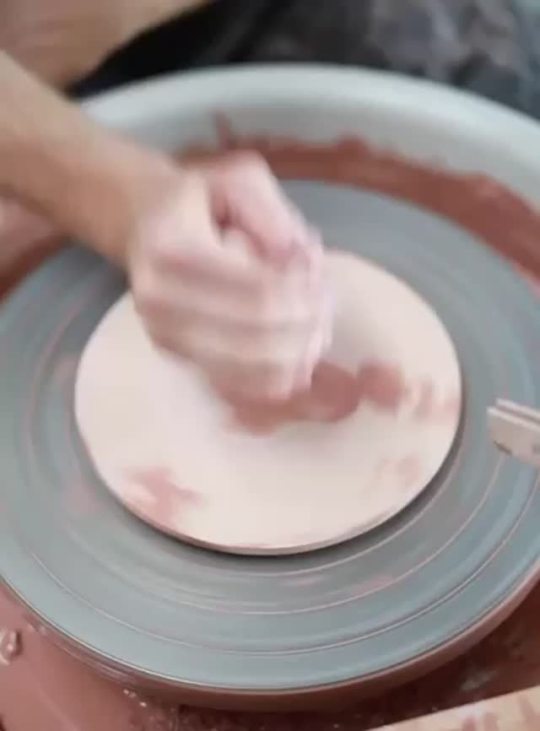The image captures a person working at a pottery wheel, with a slightly blurry and indistinct background. In the upper right-hand corner, there is a black blur. The overall blur affects the clarity of the scene. From the upper left-hand corner, there is a hand extending towards the center of the wheel; the hand appears blurry and is clenched into a fist. The fist is positioned centrally on the wheel, which is gray with light lines. Beneath the fist, a light tan circle is visible, accentuating the central focus. The wheel itself features a darker brown hue outside the tan circle. A white, plate-like disc lies centrally on the pottery wheel, and below it is a blue disc. Further beneath, there's a darker brown substance, possibly clay, suggesting a pottery process in progress.

The colors in the image include shades of peach, tan, brown, white, blue, black, and off-white. Although the exact setting is ambiguous, it hints at either a home environment or an art studio, serving as a versatile backdrop for the pottery activity. The composition positions the fist and the nested plates centrally, indicating a focus on the tactile interaction with the pottery material, albeit the clay is partially obscured or enclosed within the clenched fist.